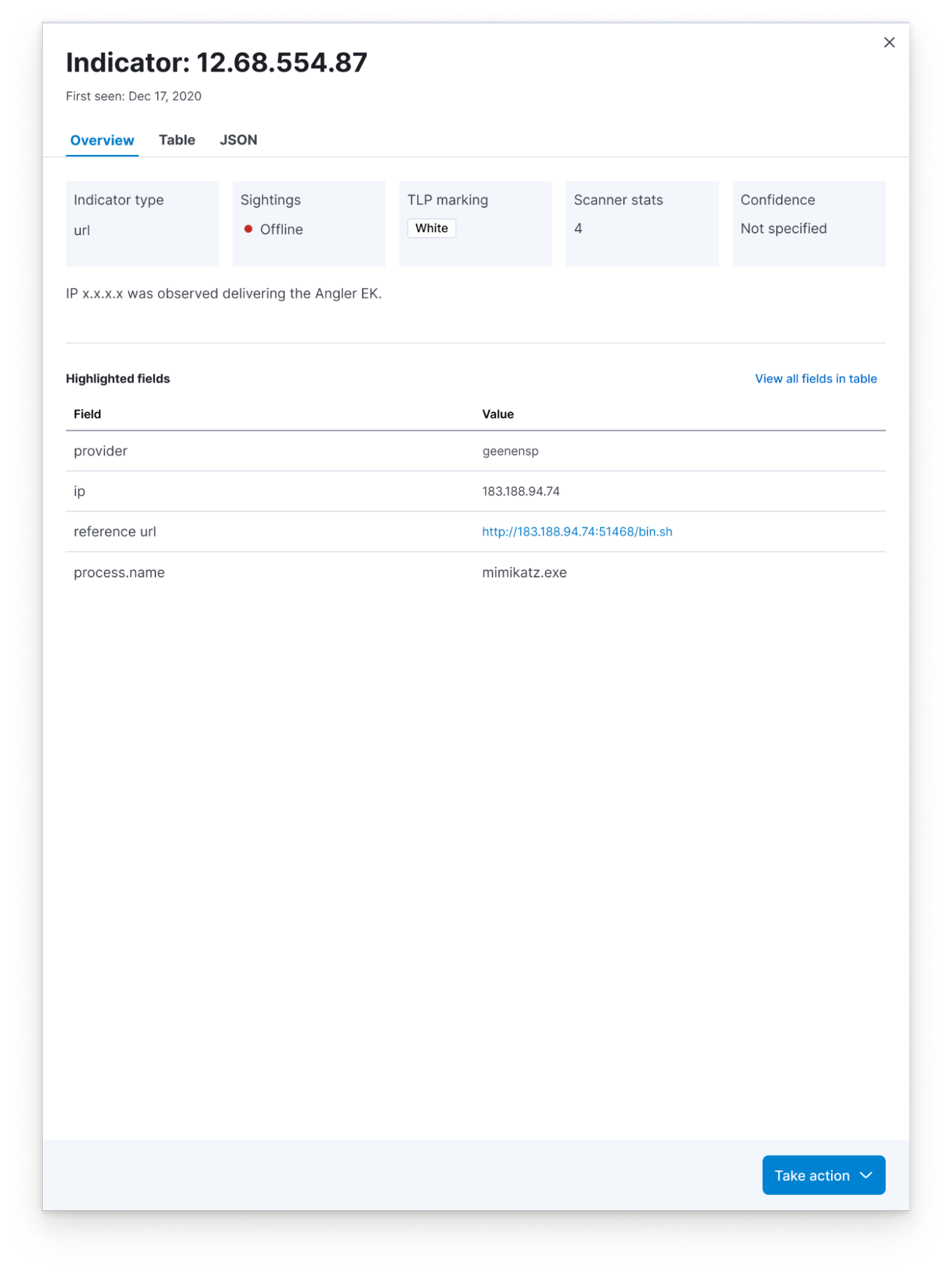A detailed screenshot showcasing an information page titled "Indicator" prominently at the top, followed by a series of numbers separated by periods. Directly beneath the indicator number, in small text, it reads "First Seen," accompanied by a specific date. The page is divided into multiple sections. The topmost section features three selectable result options: "Overview," "Table," and "JSON." The "Overview" option is selected, highlighted with blue text and an underline.

Below these options, five horizontally-aligned fields are visible, each in a light blue rectangle: "Indicator Type," "Sightings," "TLP Marking," "Scanner Stats," and "Confidence" with varying values inside them. Underneath these fields, there is a generic IP notation indicating "IP x.x.x.x was observed delivering the Angler EK," separated by a thin horizontal line.

In a darker font, the section titled "Highlighted Fields" is prominent at the top. Opposite to it, in blue highlighted text, is the phrase "View All Fields In Table." Directly below this line, two columns are present: "Field" and "Value." The "Field" column lists "Provider IP," "Reference URL," and "Process Name" over four lines. Correspondingly, the "Value" column displays "gene ENSP," a numerical value with periods, a URL address, and "mimikatz.exe is executable."

A third, currently empty, column titled "View All Fields In Table" is positioned adjacent to these. Located in the bottom right-hand corner, a small blue button labeled "Take Action" with a drop-down arrow is visible, providing further interaction options.